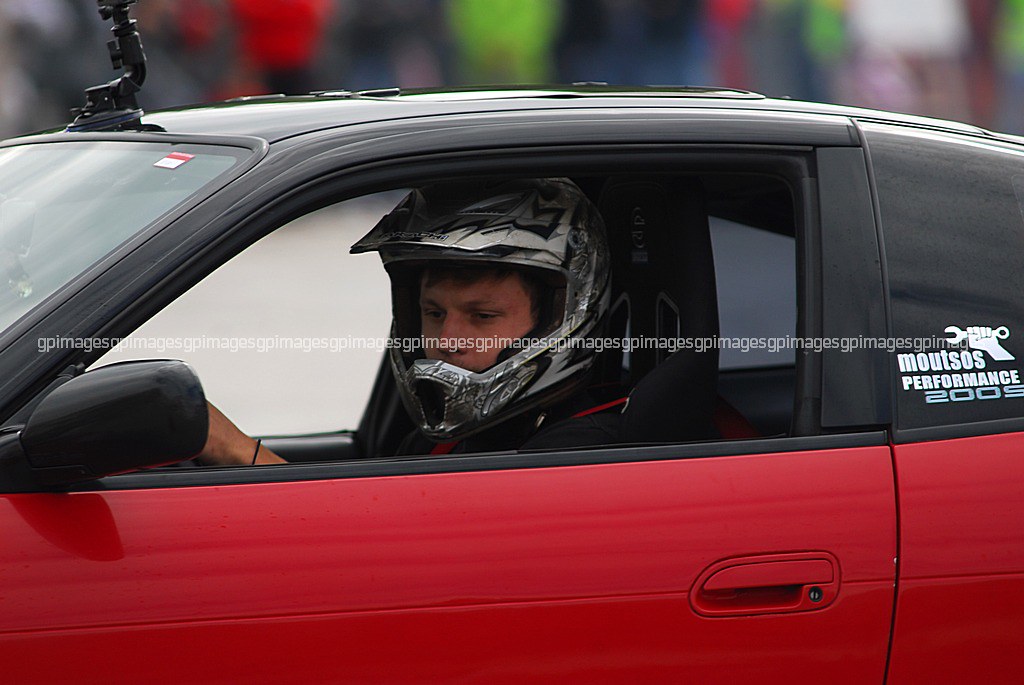The image features a detailed close-up of a focused driver sitting in a red rally or sports car at a racing event. The driver, who has light-colored skin resembling the actor Michael Cera, wears a distinctive black helmet with a chin piece, similar to a motorcycle or professional racing helmet. The red vehicle, identified by the visible driver’s side door and rolled-down window, sports a black top and a large logo on the side reading "Mutzos Performance 2009," accompanied by a white graphic of a hand holding a wrench. Positioned to the left of the frame, the car faces leftward and is surrounded by a blurred background with hints of spectators, indicating the high-energy atmosphere of the event. The image also has a repeated watermark reading "GP Images," emphasizing its official nature. An affixed object is visible atop the car, suggesting additional equipment or modifications consistent with racing.